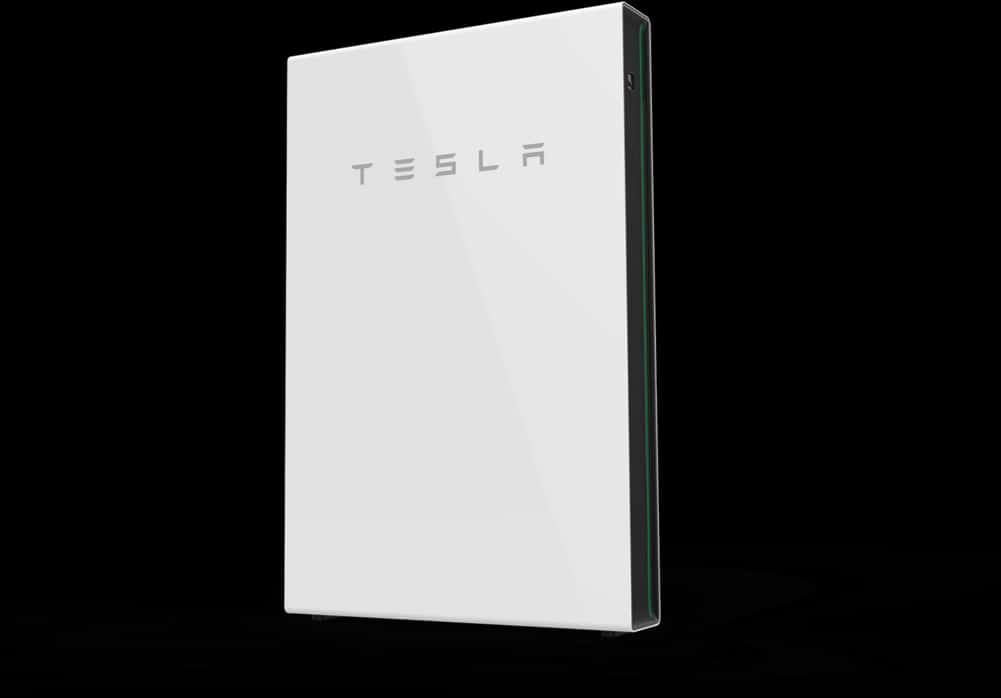A sleek, computer-generated image features a white, ultrathin rectangular box set against a solid black background. The box, longer on the horizontal axis, is viewed from both the front and side, accentuating its narrow profile. Positioned in the upper third of the box's front face is the bold, uppercase text "TESLA." To the right, the box reveals its black interior within the white shell, accentuated by a vibrant green line running vertically along its edge. On the top left corner of the box, a smaller black rectangle is visible, potentially housing a toggle switch, though its details are somewhat indistinct. The image appears highly polished and smooth, devoid of pixelation, and floats prominently in the center of the frame. Notably, the upper right corner of the box reaches the frame's top edge, tilting inward and leaving all other sides free from contact with the frame's borders.